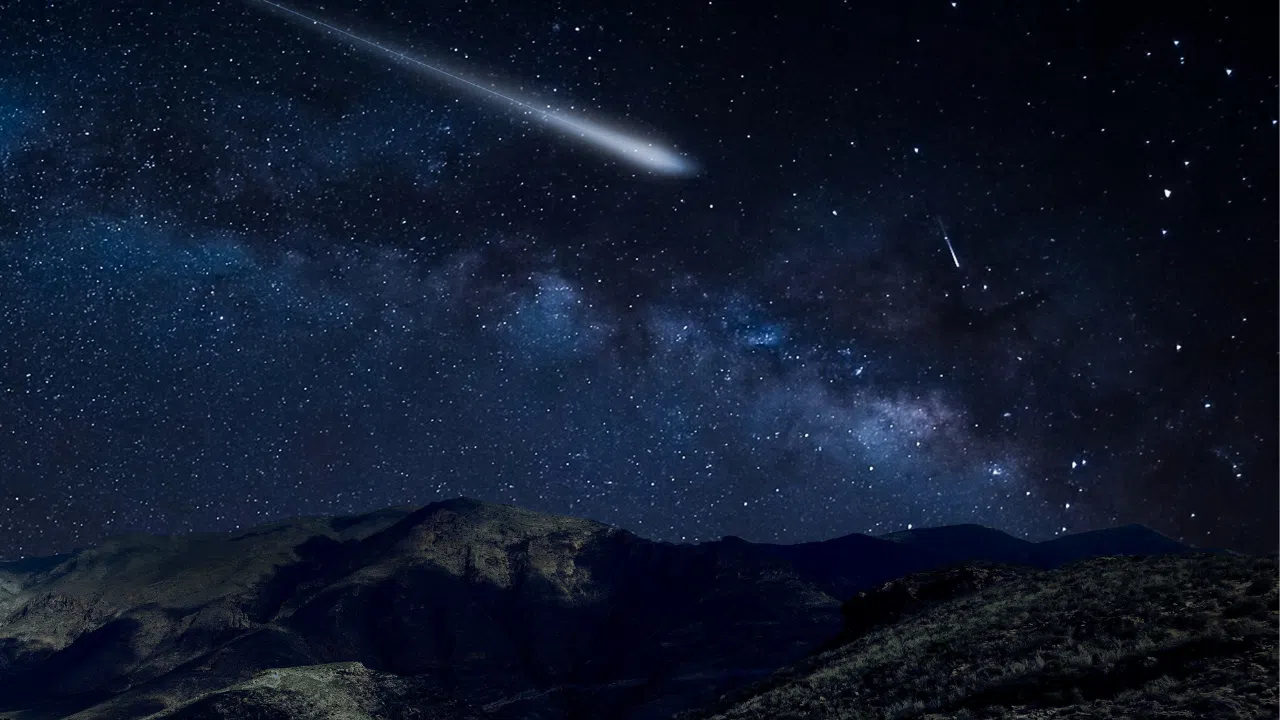The photo captures a breathtaking, expansive view of a starry night sky, observed from a rugged, hilly mountainside. The ground, occupying the lower third of the image, is devoid of trees and stretches out in rough, dark silhouettes against the night. Above, the sky radiates in a gradient of dark and rich blue shades, transitioning to almost pure black in the upper right corner. The entire celestial canvas is generously sprinkled with countless stars. Prominently, there's a dynamic streak cutting through the upper left portion of the image, possibly a shooting star or comet, trailing swiftly across the sky. The center of the sky appears to hint at the edge of a galaxy, adding a profound depth to the scene. The overwhelming stillness of the scene, punctuated by the luminous star-studded sky, evokes a sense of awe and tranquility.